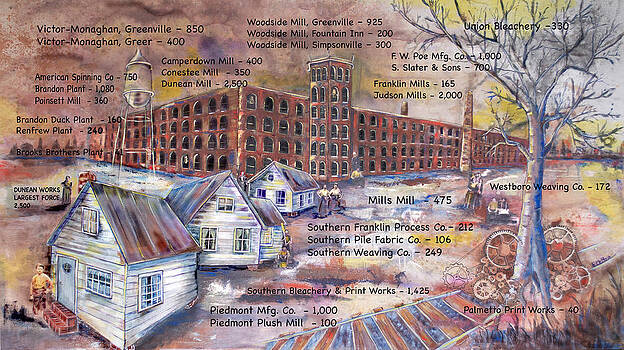This detailed artist's rendering, possibly a watercolor painting, showcases an expansive commercial or industrial area from around 100 years ago. The focal point is a prominent four-story brick building, extending across the image, with a central tower that adds an additional two stories. Labelled as Franklin Mills, Judson Mills, Camperdown Mill, Comstock Mill, and Dunedin Mill, this structure likely represents various manufacturing spaces. In front of the building, three small white houses with A-frame roofs are depicted, one of which has a boy in yellow standing by its brick steps. Further elements include a barren tree on the left, near some railroad tracks, and bicycles parked under another tree on the right. The background features slightly taller buildings and extensive written labels and numbers, such as Victor Monaghan Greenville 850 and American Spending Company 750, which appear to detail the capacities or employment sizes of various factories. Small images of people are scattered around, enhancing the bustling ambiance of this historical commercial hub.